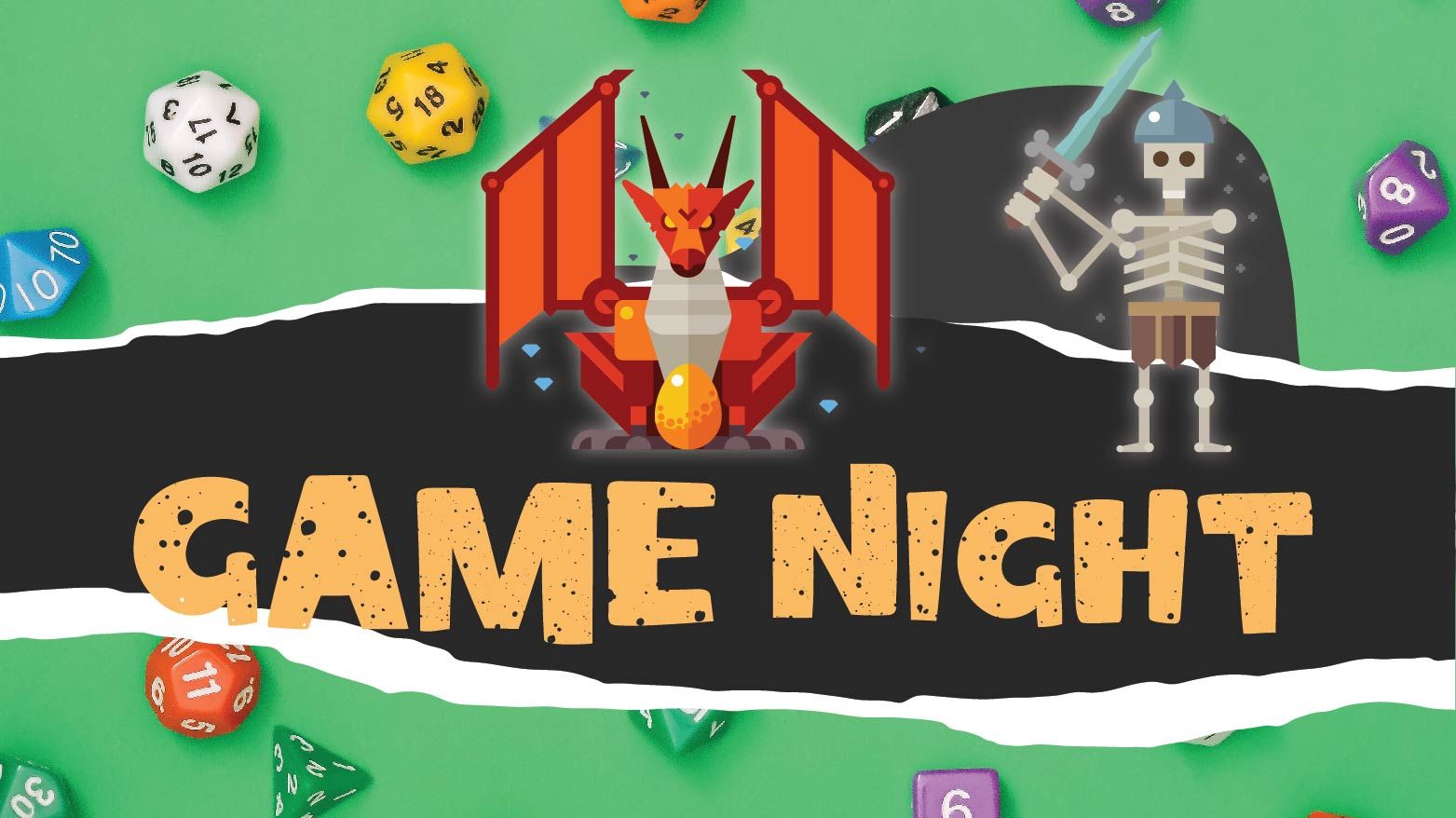The image appears to depict the start screen of a computer application for game night selections. The background is a large, vibrant green rectangle populated with various polyhedral dice, including 4-sided, 5-sided, 6-sided, and 16-sided dice. At the center of the screen, there is an old-school, pixel art-style dragon, adding a nostalgic video game feel. A skeleton dressed in brown pants is also featured in the scene, dynamically swinging a sword. Dominating the image is a bold text that reads "Game Night," displayed above a black banner stretching horizontally across the screen. This setup suggests that the app provides a variety of games to choose from, enhancing the excitement of game night.